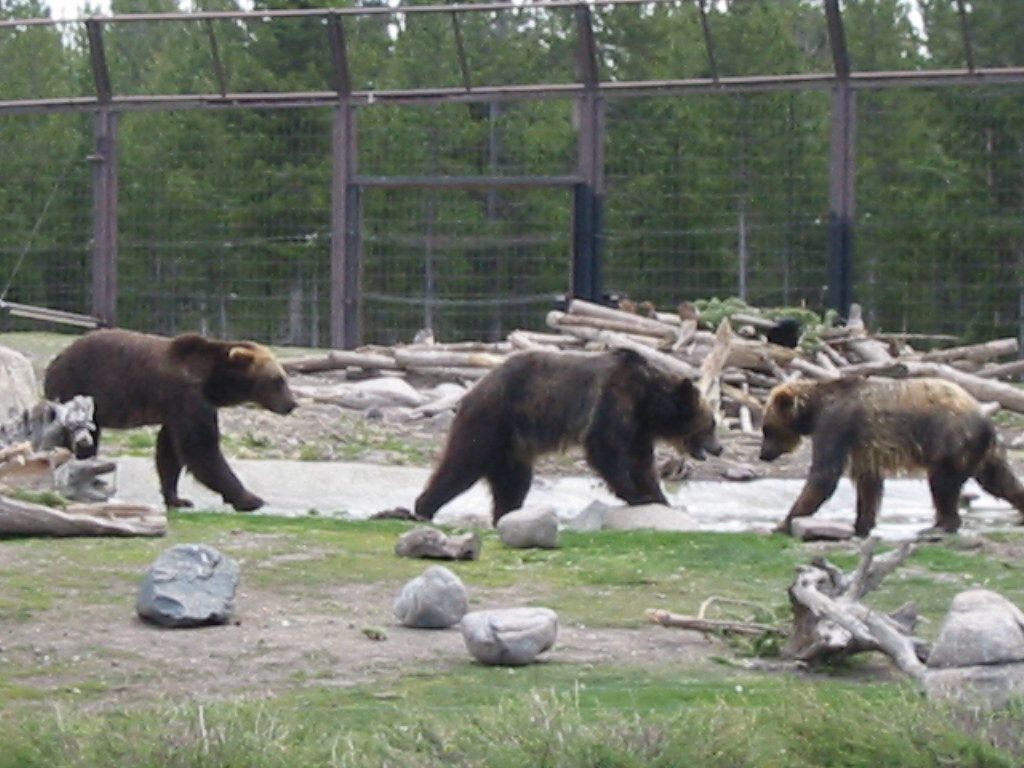The photograph depicts a zoo or similar animal enclosure surrounded by high, brown, metal bars and chain-link fencing, which extends over the top, creating a complete enclosure. Inside, three brown bears are visible; two are walking toward the right, while one smaller, lighter-colored bear is moving to the left, with its mouth open, possibly interacting with the other two. The bears are on a gravel walkway within the enclosure. The foreground includes a grassy area interspersed with dirt and large stones, with a piece of driftwood resting on top. In the background, there are some trees and a significant pile of wood, comprising tree stumps and branches.